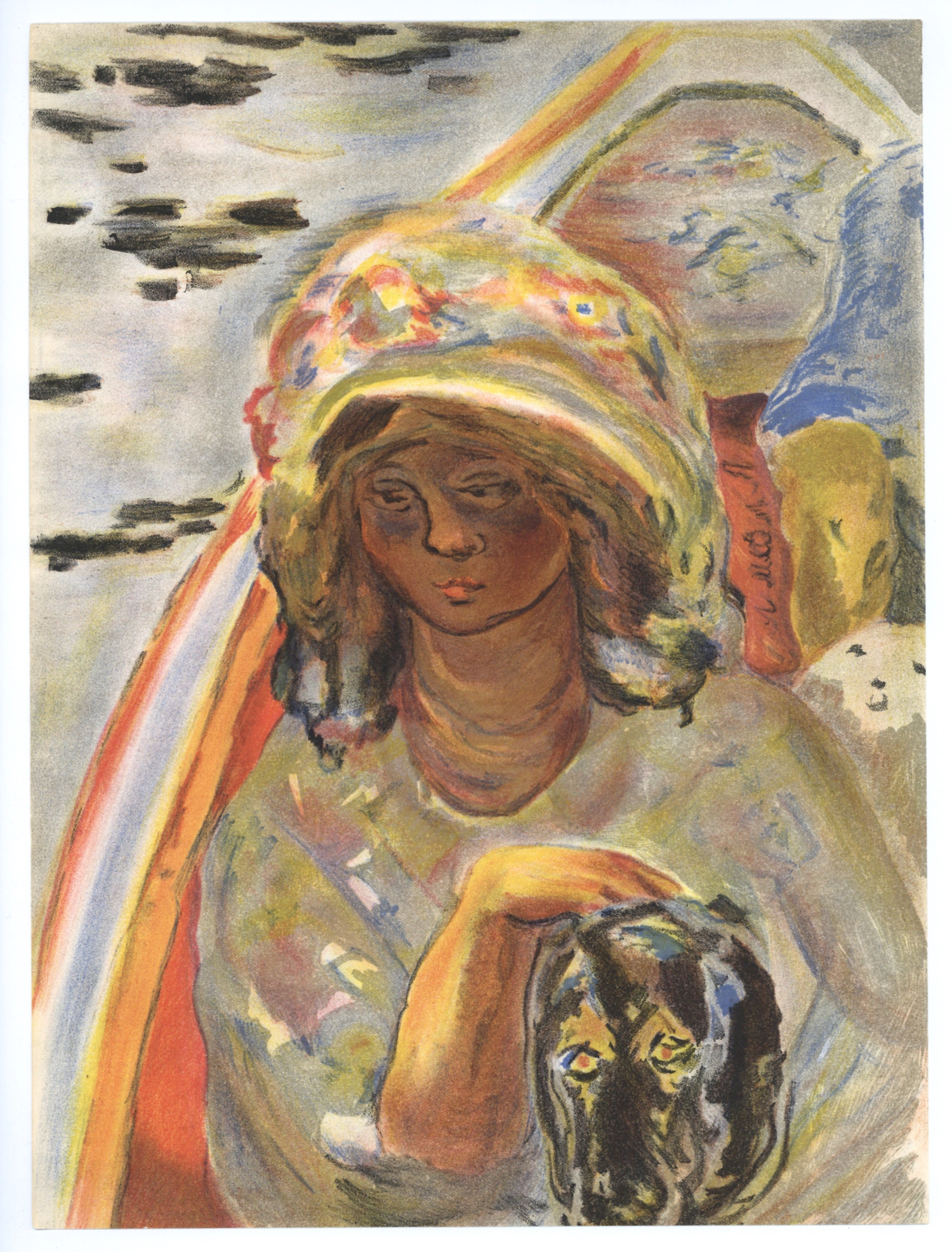The painting is an abstract, hand-painted image of a contemplative woman with beige-colored skin and blondish, brown hair, dressed in a white dress with blue and yellow patches. She is wearing a yellow, brimmed hat adorned with a floral pattern, which slightly covers her hair. The woman is sitting in a small boat with green water in the background that features lime and olive green tints. Her elongated neck and pensive expression suggest a sense of sadness or deep thought as she looks down toward the left of the picture. 

The woman has her arm around a black Labrador-like dog, petting its back with her right hand. The dog’s face is adorned with blue, red, and yellow highlights, adding to the painting’s vibrant color scheme of beiges, yellows, browns, and sparse reds. The boat is depicted with a light wood-colored gunwale and a wooden hull, suggesting a natural and serene setting.

In the background, lily pads float near the boat, with reflective water featuring cloud-like light patterns, adding depth and tranquility to the scene. There's an orange-colored bag near the woman’s hand, along with some indistinct objects in the rear of the boat. The background also contains faint black splotches and possibly more reflective water elements, enhancing the painting's abstract nature.